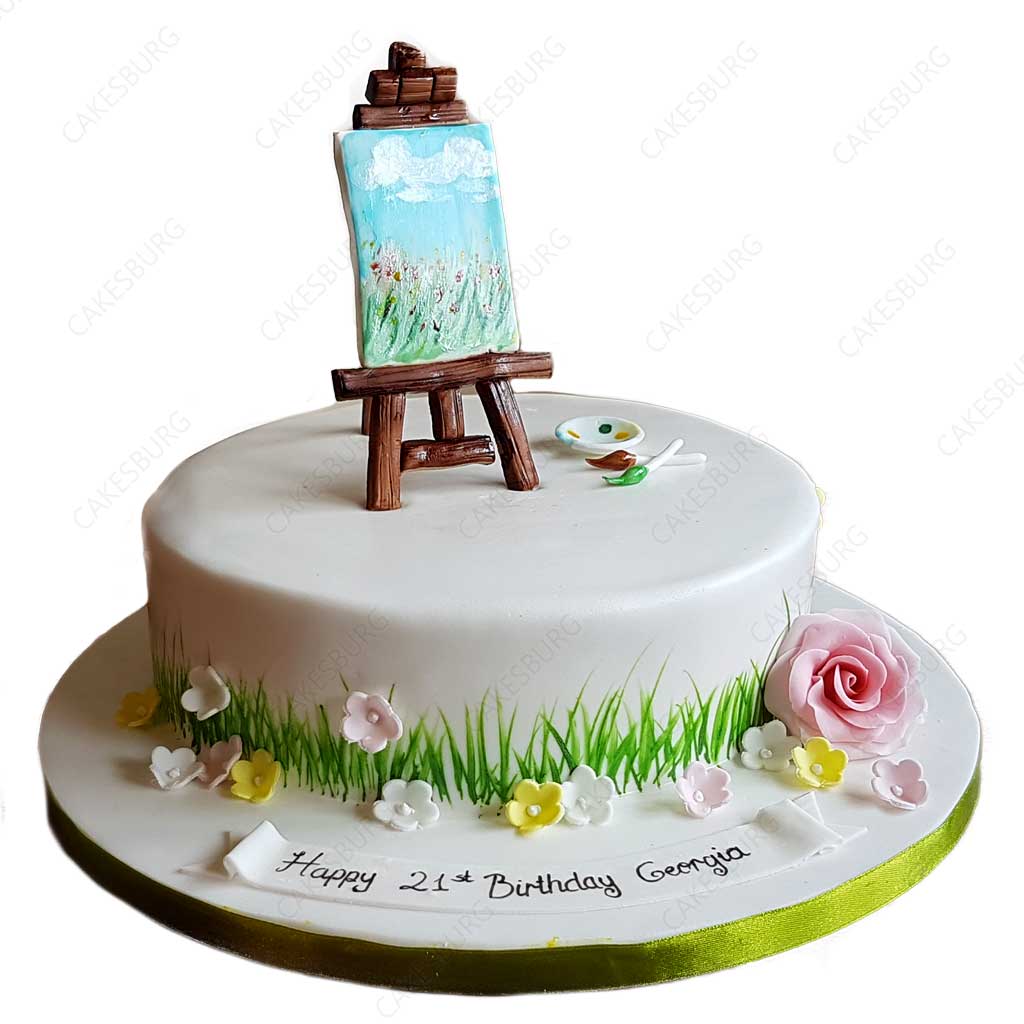This image is a color photograph of a meticulously decorated, one-layer fondant birthday cake against a white background. The cake is adorned with green blades of grass painted around its smooth white sides. Scattered among the grass are fondant flowers in white, pink, and yellow, with one prominent pink rose on the right side. Atop the cake sits a brown wooden easel, crafted from fondant, displaying a painting of a grassy field under a blue sky with white clouds. Beside the easel rests a paint palette with two paintbrushes, one tipped with green and the other with brown, both featuring white handles. The cake sits on a white base wrapped in a shiny bright green ribbon. Inscribed in elegant black cursive fondant along the base are the words, "Happy 21st Birthday, Georgia." The detailed cake design suggests it was made for someone who is an artist or has a fondness for painting.